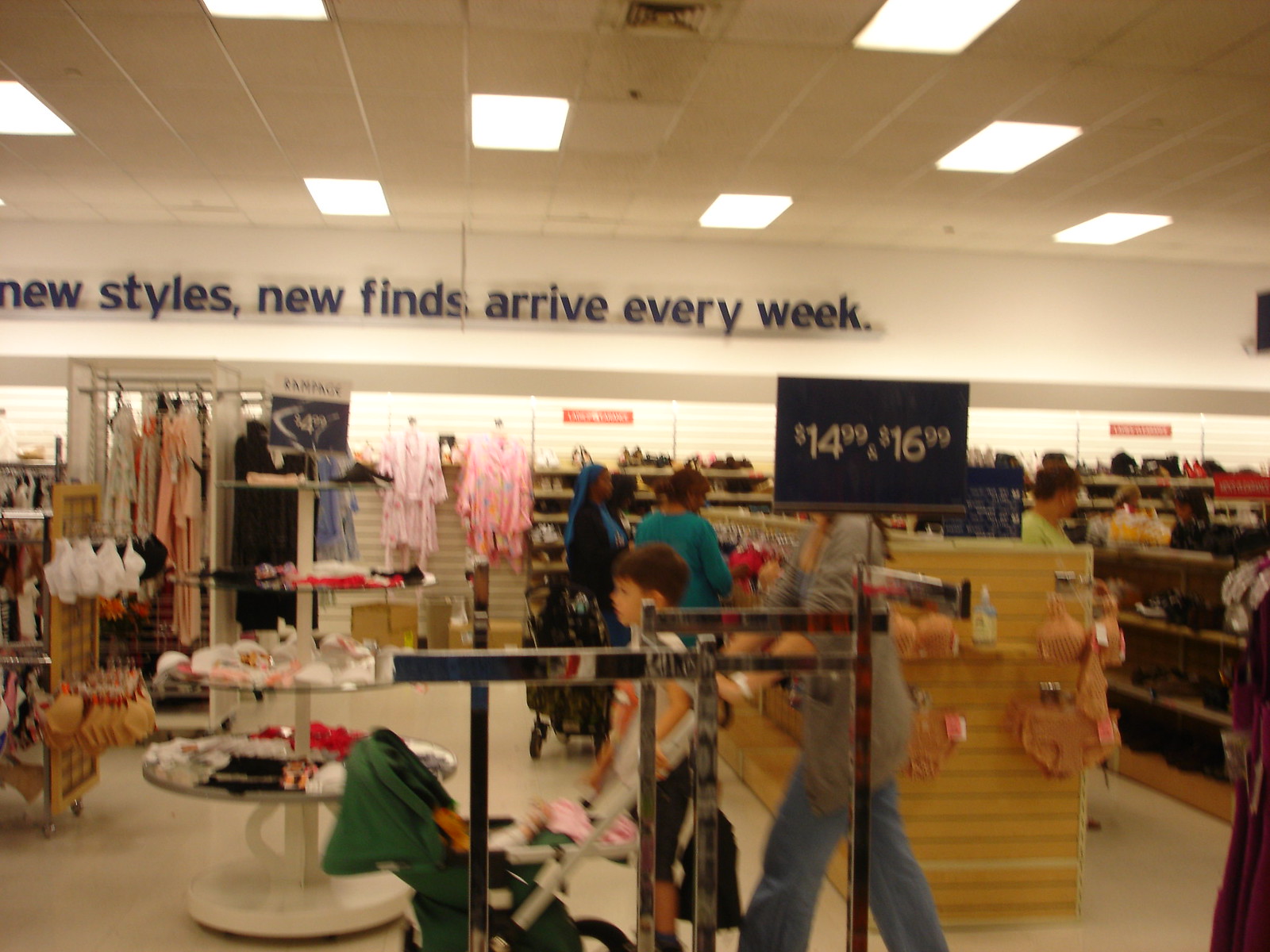This photograph, taken inside a bustling department store, captures a moment in the women's clothing section. The store features white walls and a typical white tile ceiling, some of which house halogen light sources with plastic coverings. Prominent on the white walls are blue letters spelling out, “New Styles, New Finds, Arrive Every Week.” The foreground of the image prominently displays an empty, reflective chromed clothing rack topped with a blue rectangular sign advertising prices ranging from $14.99 to $16.99. Just behind this rack stands a woman wearing a gray shirt and blue jeans, pushing a green stroller with white handles, accompanied by a little boy dressed in a white shirt and black shorts. The blurry depiction suggests that there are various shoppers in the background. The store layout includes large aisle dividers featuring women's lingerie and shoes, and the background shows ridged walls designed for hanging clothing, some adorned with bathrobes. This scene encapsulates the typical hustle and bustle of a department store's women's clothing area.